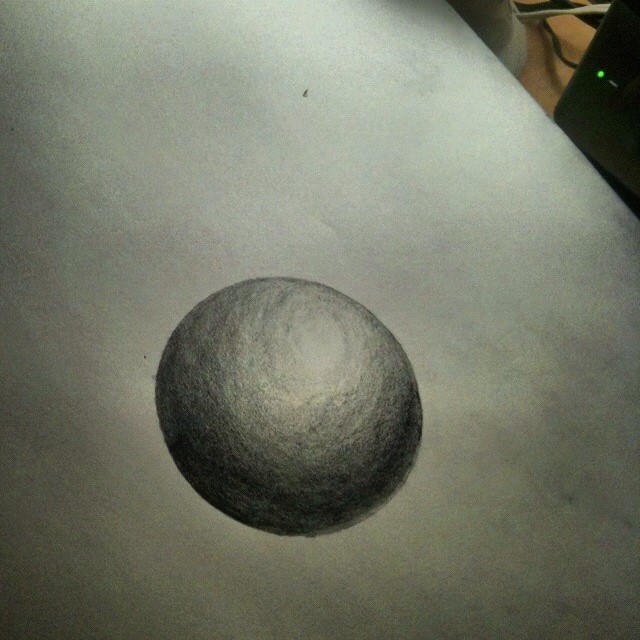In this black and white photograph, an intricately detailed charcoal or pencil drawing of a sphere is displayed on a white table with a subtle grayish background. The sphere is meticulously shaded, with the darkest tones at the bottom graduating to lighter tones toward the top, creating a convincing 3D effect. The sketch captures even the smallest imperfections, enhancing its realistic appearance. Adjacent to the drawing, on a light brown table surface, sits a black device, likely a modem, marked by a small green indicator light. This modem is connected by a black plug and accompanied by another white wire leading to an unspecified device.